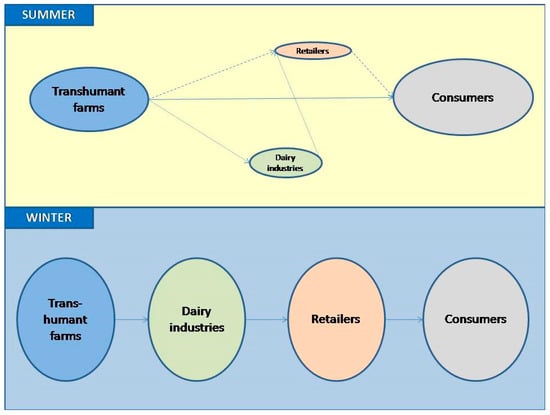The image is a detailed visual aid divided into two halves, representing concepts of "Summer" and "Winter." The top section, which has a yellow background, features a blue rectangle at the top left labeled "Summer" in yellow text. Within this section are four oval shapes of varying colors and sizes. On the left, a large blue oval is labeled "Transhumant Farms" in black text. To the right, there's a large purple oval labeled "Consumers," while in the middle, two smaller ovals are positioned one above the other: a pink oval at the top labeled "Retailers," and a green oval at the bottom labeled "Dairy Industries." These ovals are interlinked with arrows indicating the direction of interaction and connection among them.

The bottom section, with a blue background, mirrors the top section’s theme but is labeled "Winter" in the top left corner. In this section, four evenly sized ovals are arranged horizontally from left to right. The color scheme from left to right includes: blue for "Transhumant Farms," light green for "Dairy Industries," pink for "Retailers," and gray for "Consumers." Each oval connects to the next with arrows, representing the flow of interaction through the winter season.